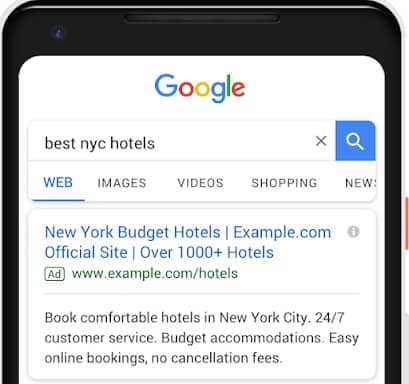The image showcases the outline of a smartphone prominently displaying its black border and distinctive elements such as the camera lens on the left side and a large rectangular speaker bar at the top center, where a reflective shine highlights the top edge of the phone.

On the phone's screen, a Google search page is clearly visible. At the top of the screen, the familiar Google logo rests against a white background. Directly beneath the logo is a search bar containing the query "Best NYC Hotels." To the right of the search bar, an "X" icon and a blue search button are easily identifiable.

Below the search bar, a navigation bar provides options to filter search results by web, images, videos, shopping, and news. Moving further down the page, an ad appears, highlighted in blue font, promoting "New York Budget Hotels" with the URL example.com, designated as an official site offering over a thousand hotel options. The ad's caption reads, "Book Comfortable Hotels in New York City, 24-7 customer service, budget accommodations, easy online booking, no cancellation fees," providing a concise but informative description of the services offered.